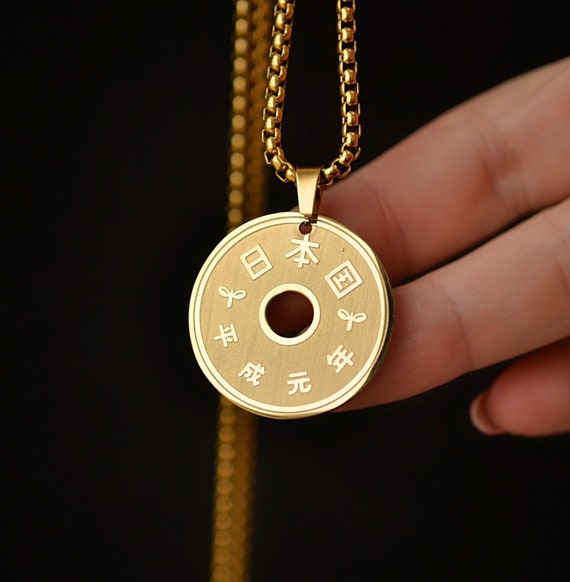In this high-resolution, sharply-focused close-up photograph, a woman's manicured hand is delicately holding a pendant made from a Japanese coin, suspended on a gold box-style chain. The pendant, light gold in color, features intricate designs and characters including traditional Japanese symbols and what appear to be tied tassels. A drilled hole at the top of the coin is fitted with a tiny gold bail, seamlessly attached to the chain. Only three of the woman's fingers are visible, with a prominently long nail on her pinky finger, which articulates a sense of elegance. The rich details of the pendant and chain stand out vividly against the plain black background, emphasizing the lustrous textures and fine craftsmanship of the jewelry.